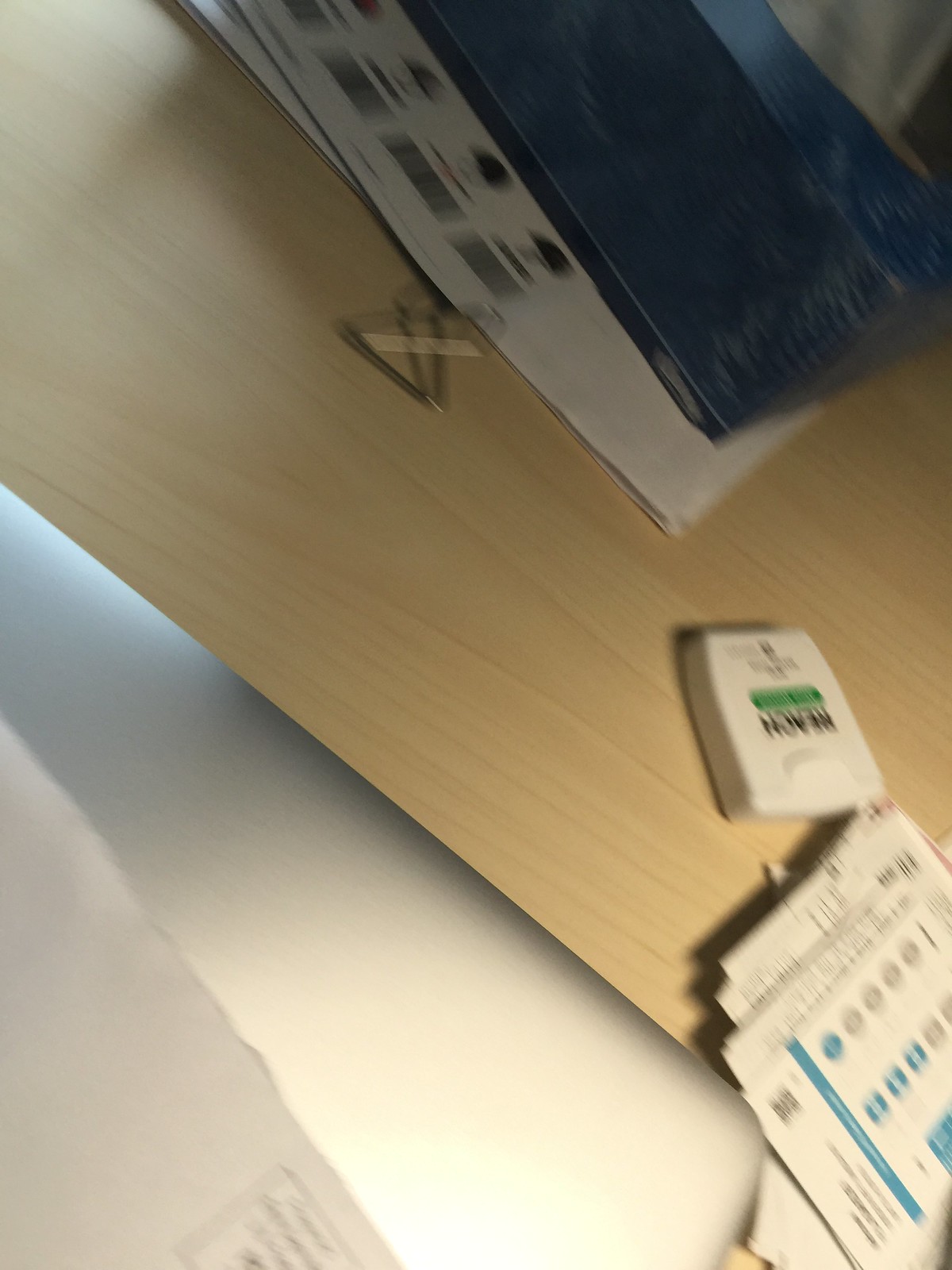The photograph, slightly blurry and taken at an angle indoors, features a tabletop crafted from wooden planks. Positioned on the tabletop is a blue box of Kleenex tissues. To the lower right, there is a square white plastic container of Reach dental floss, easily identifiable due to the green line under the brand name. Surrounding the dental floss, there is a jumble of white paper, likely mail or receipts, some of which bear black writing and blue icons. Among these papers is a stack that might contain prescriptions, as indicated by the blue dots on some sheets. Additionally, there’s a silver clip or possibly the corner of a MacBook, along with a metal paperclip. Beneath these objects, one can also spot a piece of mail displaying a prepaid postage stamp. The image being out of focus does make it challenging to discern finer details, but the key elements—a blue Kleenex box, Reach dental floss, scattered papers, and various office supplies—are clearly visible.